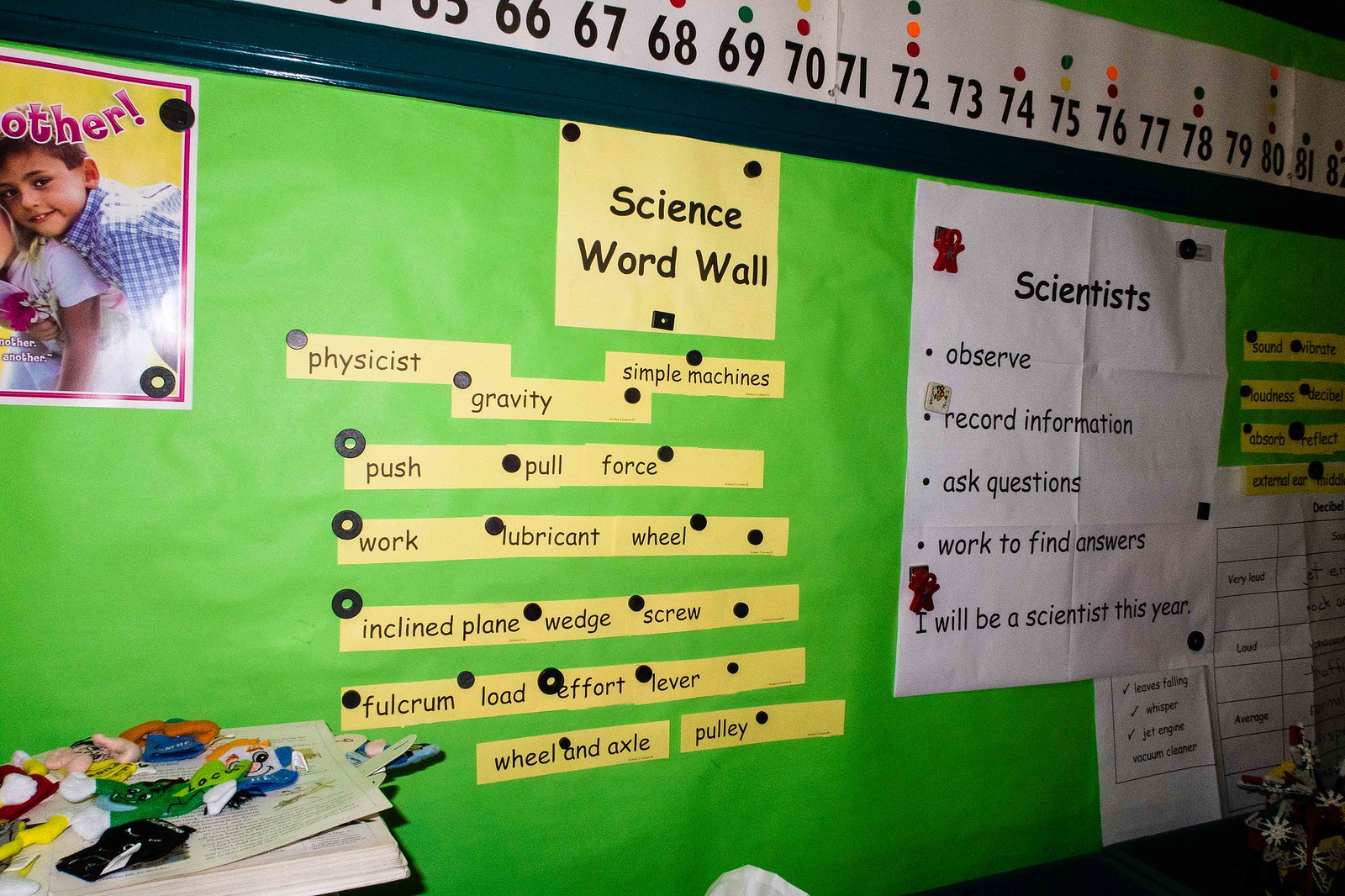This image depicts a classroom bulletin board prominently featuring a science-themed word wall designed for young students. The board is covered in lime green paper, with a white banner at the top displaying partially cut-off black numbers ranging from 65 to 82. A central poster illustrates a small boy and girl, accompanied by an orange banner reading "Science Word Wall." Beneath this, neatly arranged yellow rectangles with black text list various scientific terms: Physicist, Gravity, Simple Machines, Push, Pull, Force, Work, Lubricant, Wheel, Incline Plane, Wedge, Screw, Fulcrum, Load, Effort, Lever, Wheel and Axle, and Pulley. Additional yellow rectangles present vocabulary words like Sound, Loudness, Absorb, External Ear, Vibrate, and Decibel.

To the side of the word wall, a white piece of paper with black text outlines core scientific principles: "Scientists: Observe, Record Information, Ask Questions, Work to Find Answers. I will be a Scientist this year." The background consists of a large roll of green paper acting as a canvas for these educational elements. In the foreground, a table holds race cars painted in various colors—black, green, blue, white, red, and yellow. The overall setup is a vibrant and educational display aimed at teaching and inspiring young learners about the fundamental concepts of science and the scientific method.